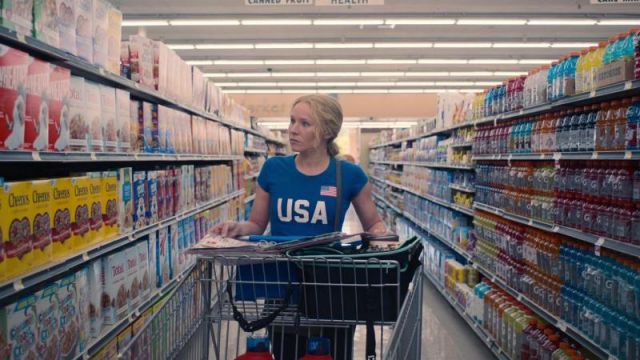The image appears to be a screenshot from a TV show or movie, featuring a blonde woman with light skin and her hair in a ponytail, shopping in a grocery store. She's wearing a blue shirt emblazoned with "USA" in large white letters and a small American flag above the "A". She is pushing a cart with a headband stretched across the top and multiple blue bags inside. She holds an open magazine or map atop her cart. The aisle she is in has shelves stocked with various cereals, including a prominently placed Wheaties box featuring Serena Williams, to her right. On her left, the aisle is lined with energy drinks like Gatorade and Powerade. The store has bright, flaccid lighting fixtures above, and windows indicating it's daytime outside.